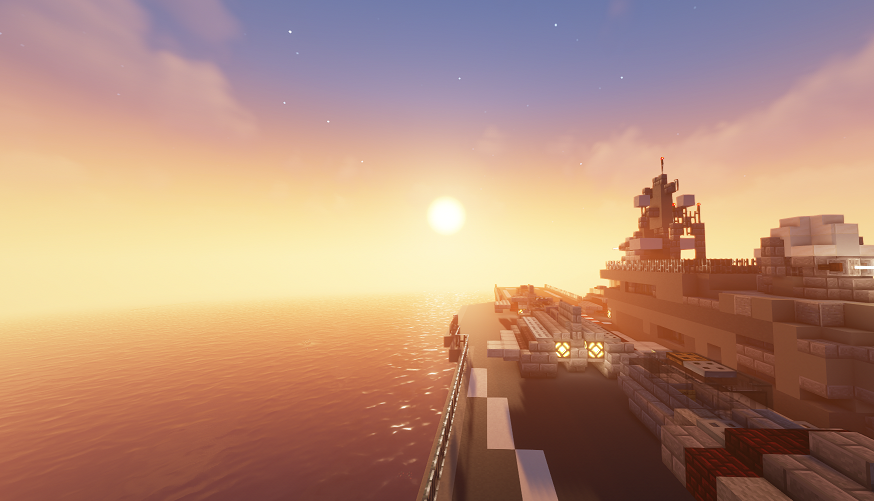This is a horizontal rectangular image, possibly from a video game with a blocky, Minecraft-like texture. The central focus is a large container ship on the lower right side of the photo, stacked with dozens of large brightly colored containers. The scene takes place outdoors, either very close to sunrise or sunset, and is cast in a vivid palette of intense oranges and yellows from the setting or rising sun near the horizon. Most of the image is dominated by the sun, a bright circle almost touching the water, which reflects its golden hues. Above it, the sky transitions to a clear blue with scattered clouds and a few white dots that might suggest stars. The ocean beneath the sun is relatively calm, displaying an orange tint. This rendered scene captures a serene and expansive maritime atmosphere.